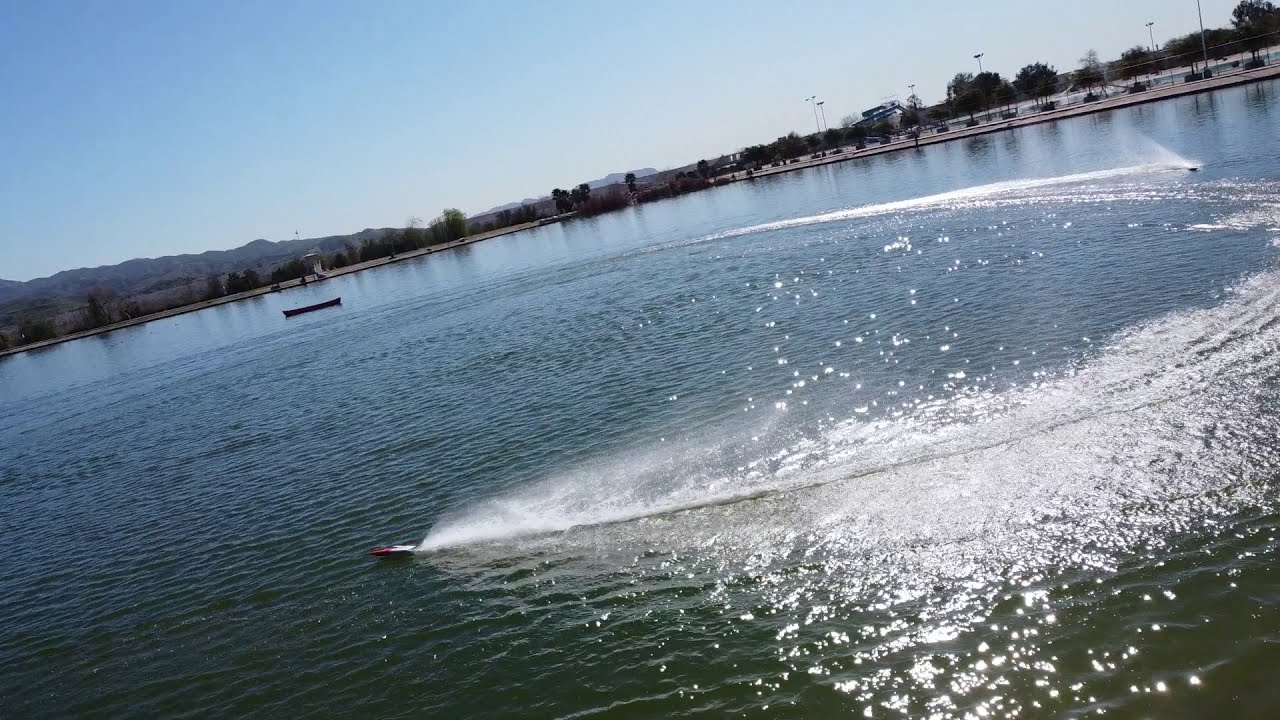This photorealistic image captures a scenic lakeside view with a dynamic composition. The photograph, taken during the daytime, is slightly tilted left, creating an off-kilter perspective. The camera captures a vast lake that spans the frame, its waters transitioning from blue in the distance to green closer to the viewer. The lake occupies approximately the top three-quarters of the image, stretching from the right to the left corners. On the lake, two boats command attention: a prominent red and white speedboat near the center-left, trailing a large, frothy wake behind it, and a smaller, darker-colored boat near the top right, also leaving a white wake. In addition, a small canoe or boat is visible farther off to the left side of the scene.

The shoreline is dotted with green trees and occasional structures, complementing the natural beauty of the landscape. In the far distance, a rugged mountainous region rises on the left, while the sky above fades from a darker blue at the top to a lighter hue near the horizon. The sun reflects off the water surface, creating white highlights amidst the greenish-blue ripples. Further detail reveals a floating dock and what appears to be a gray brick or stone pier visible in the background, suggesting human presence and activity. The scene encapsulates a peaceful yet lively lakeside setting, likely in the midwest or mountain west region of the United States, with remote-controlled boats skimming across the water's surface, kicking up sprays of water behind them.